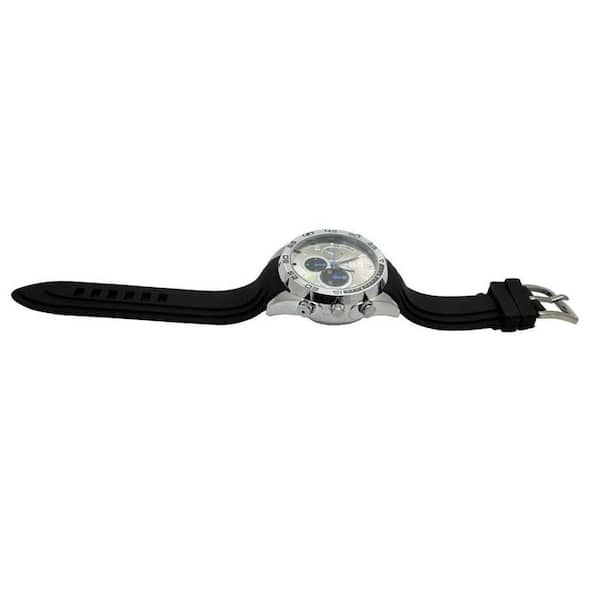The image features a wristwatch set against a completely white background. The wristwatch has a black leather strap with silver buckles. The watch, made of stainless steel, is laid sideways in the image, which makes the face somewhat difficult to see in detail due to light glare. However, the circular face of the watch is silver with small black numbers around its circumference and at least two or three smaller circles within it. The watch hands point to approximately one o'clock. The outer rim of the watch face and the underside are also silver, and there are light etchings that, while hard to read, add to its detailed design. On the right-hand side of the watch, there are two knobs, likely for adjusting the time and other functions.